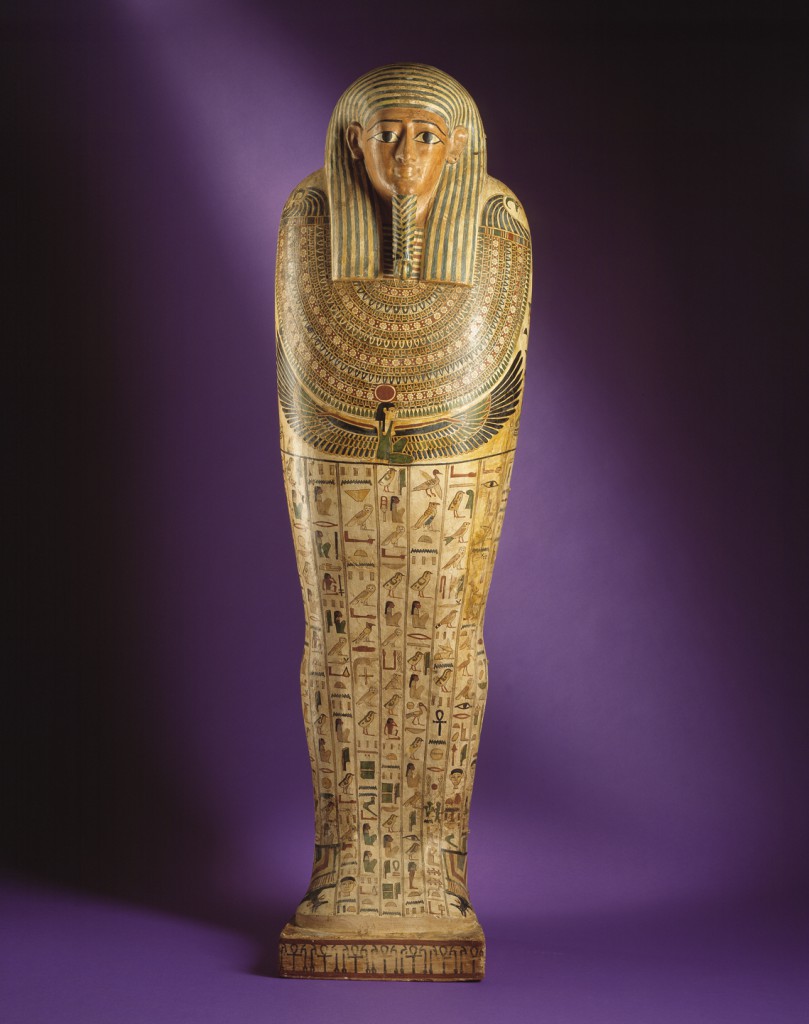This photograph captures an upright Egyptian sarcophagus, believed to be from ancient Egypt dating roughly between 332 to 302 BC, and is currently housed at the Denver Art Museum. The sarcophagus stands prominently on a dynamically lit purple background, enhancing its regal appearance. Made of gold and other vibrant colors, the case is intricately detailed and quite tall, potentially around 7 feet, although this estimation lacks a clear reference point. 

The sarcophagus features a molded face with large, expressive eyes, accentuated by black eyebrows, and the iconic Egyptian headdress flowing into long hair that reaches below the shoulders. The chest area is adorned with elaborate, curved designs and vibrant artwork patterns. Extending down to the abdomen, striking imagery emerges including a winged figure—possibly a phoenix or an eagle—symbolizing protection or resurrection. More hieroglyphs, images of birds, and other Egyptian symbols and objects decorate the remainder of the casing, enveloping the figure in a rich tapestry of ancient iconography. The base of the sarcophagus is square, and it follows the loose shape of a human body, sans limbs which would have been positioned inside the case.